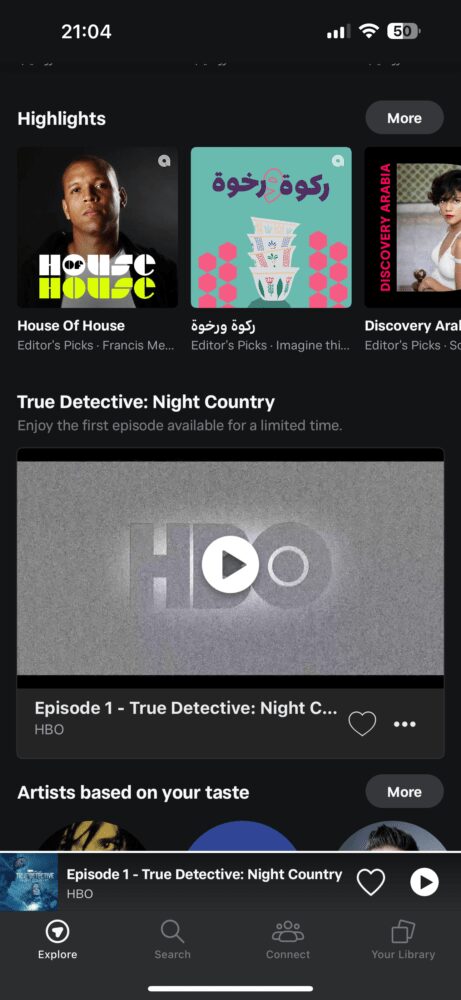The image displays a mobile device screen with a time of 21:04 and a battery at 50%, along with a Wi-Fi signal showing three bars. The screen features a heading titled "Highlights" with three thumbnails situated below it. The first thumbnail shows a person who resembles Vin Diesel, with text underneath that reads "House of House." Next to it, a caption states "Edna's Pick," followed by text partially obscured, starting with "M E..." and some text written in another language.

The third portion to the right is labeled "Discovery ARA" and also highlights "Edna's Pick." Below it, there's a promotional mention of "True Detective: Night Country - Enjoy the first episode available for a limited time," accompanied by a video with a play icon in the center and the HBO logo. Further down, it says "Episode 1: True Detective: Night Country," with another mention of HBO and a note that it is curated "Based on Your Taste."